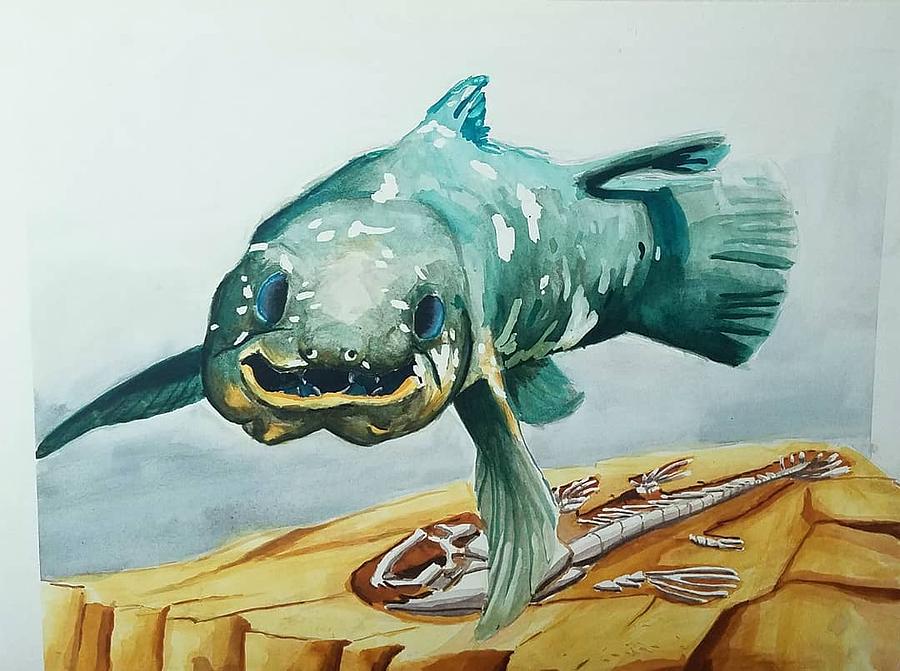This captivating image appears to be a detailed watercolor painting of a prehistoric fish presented from a frontal perspective. The fish displays vibrant blue eyes and prominent long fins, which are complemented by a sprinkling of white mottling across its predominantly blue body. The creature's anatomy includes a fin on its back arching downward, fins near its tail, and a fin on its underbelly. Its mouth is partially open with a distinct yellow edging. Notably, the painting portrays the fish mid-swim, evoking a sense of liveliness.

At the bottom of the image, a layer of tan or golden sedimentary rock, possibly sandstone, is visible, enclosing a complete white fossil of a similar fish. This juxtaposition suggests that the illustration is the artist's conception of what this prehistoric fish would have looked like when it was alive. The fossil's detailed, skeletal remains offer a stark, fascinating contrast to the imagined, vibrant portrayal of the ancient sea creature swimming above, making the image a vivid and scientifically inspired artwork.